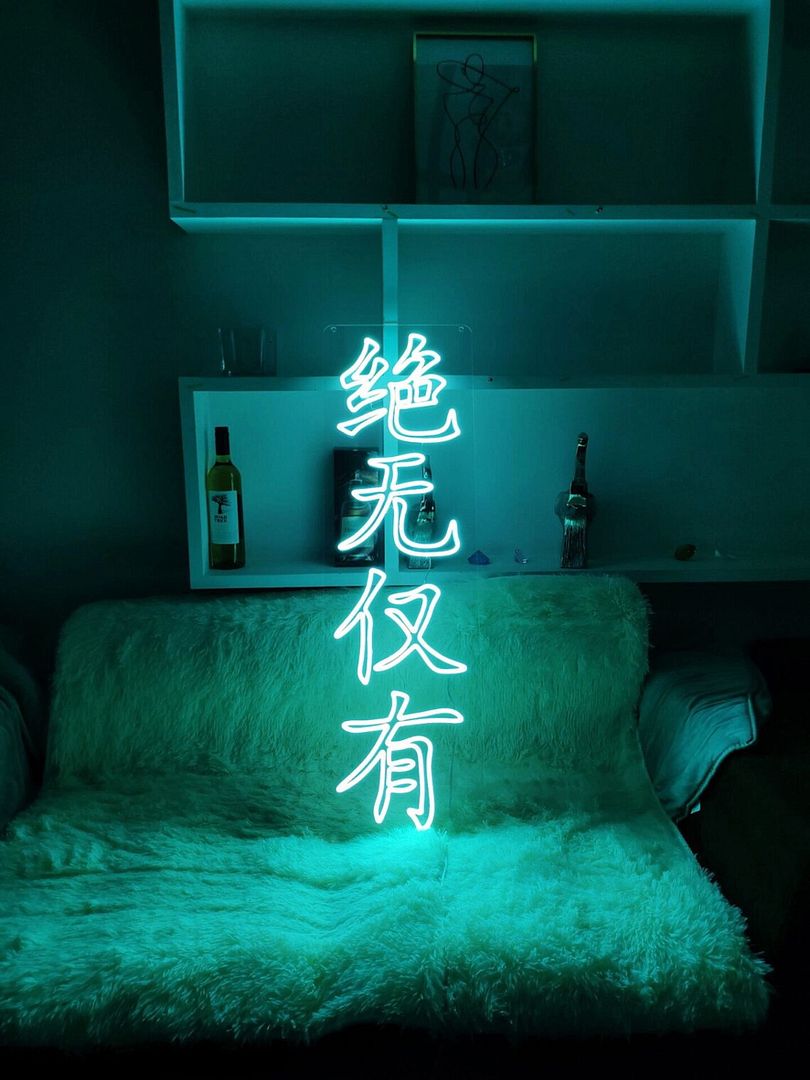The image depicts a dimly lit room with the main source of illumination being a bright blue neon sign featuring Japanese characters arranged vertically. The room primarily glows with a blue tint due to this sign, which is centrally positioned. Below the neon sign is a small sofa or large seat adorned with a white, fuzzy material, creating a stark contrast against the dark surroundings. Behind the sofa, there are cube shelves in white that hold various bottles of alcohol, including wine, along with a drinking glass. Atop the shelves, a piece of artwork resembling a sketch of an abstract human figure adds an artistic touch. The neon light not only illuminates the scene but also casts a blue-green backlight across the entire room, highlighting the intricate details and creating a cozy yet mysterious atmosphere.